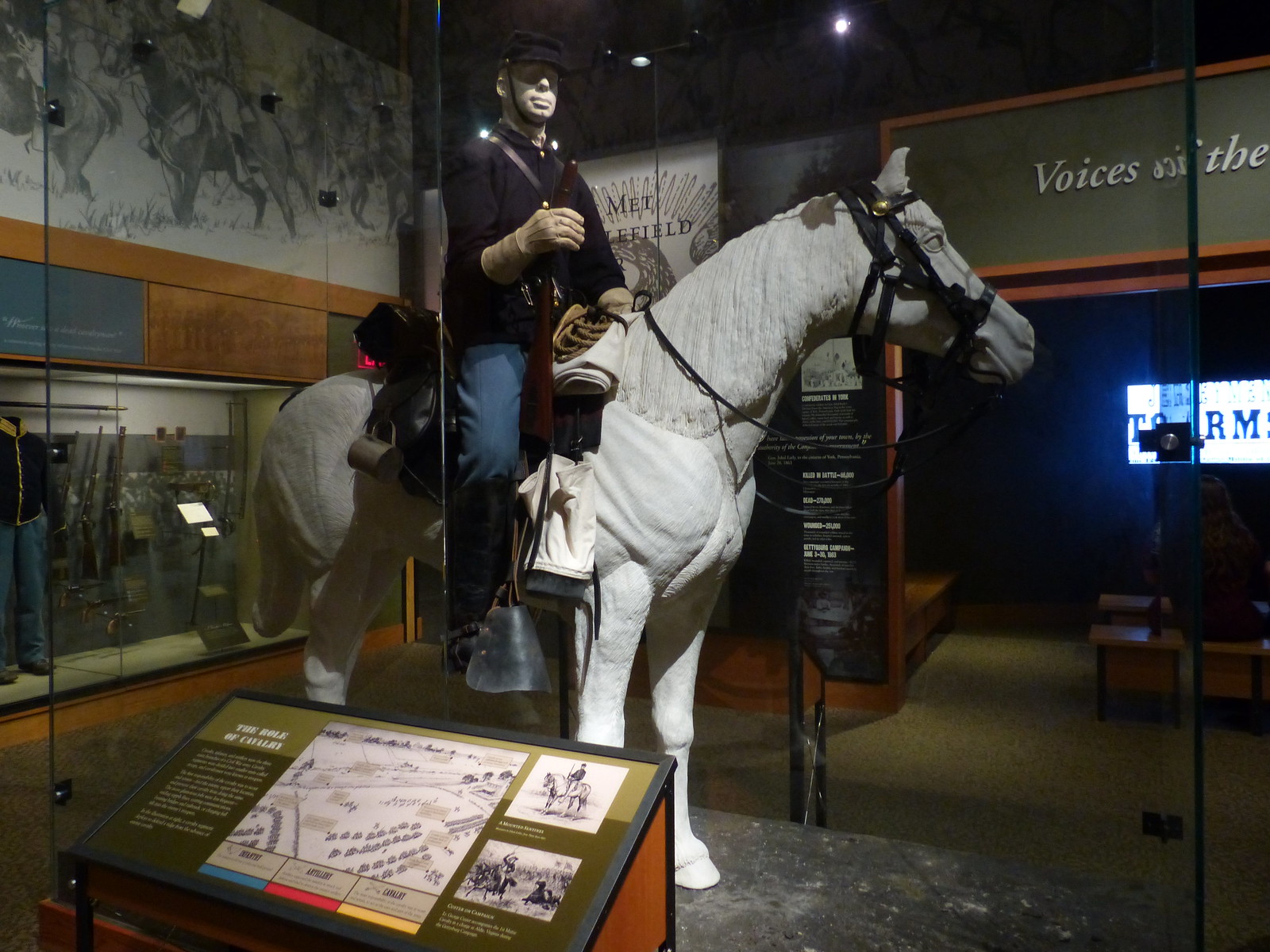The image depicts a detailed exhibit within a historical museum, likely dedicated to war history. Central to the exhibit is a striking statue of a soldier mounted on a white horse. The soldier is dressed in a Civil War-era military uniform, complete with gloves, a black top with brass buttons, a cap, and not quite navy blue pants. His hands are raised in a commanding gesture, evoking a sense of leadership and action. Surrounding the statue are various war memorabilia, including maps, guns, and a soldier's uniform encased in glass. The background features a large black-and-white painting of several people on horseback, adding depth to the historical context. Additionally, there is a detailed informational display with pictures, diagrams, and text that appears to describe the role of civilians in war, enhancing the educational aspect of the exhibit. Benches are placed in the room for viewers to sit and watch a film that further explores the historical themes presented.